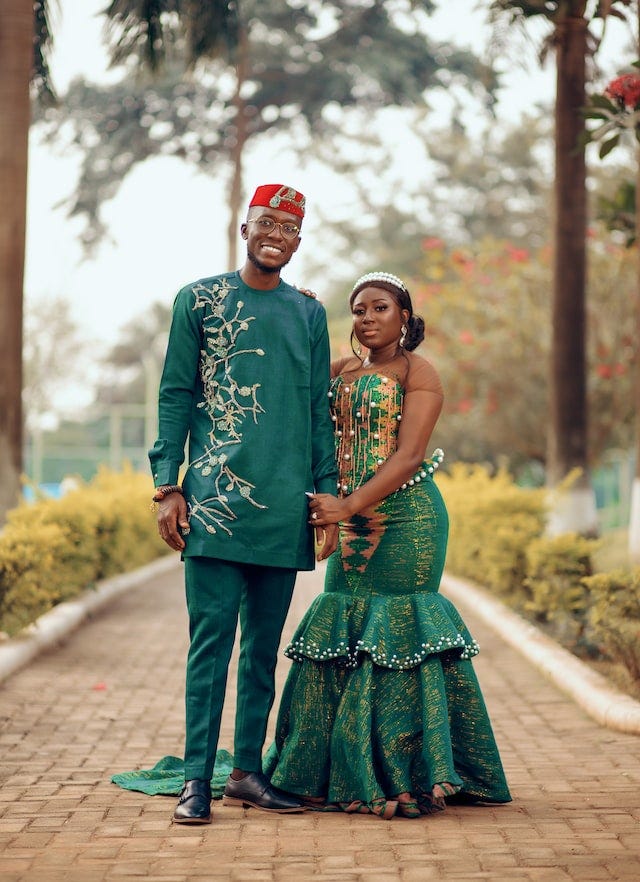The photograph depicts an afrosual couple, likely Nigerian, dressed in traditional formal attire, possibly for a wedding. The man, standing on the left, is adorned in a long-sleeved green top with intricate yellowish and beige floral embroidery on his right side, paired with matching green pants and black shoes. He sports a red embroidered fez cap and gold-rimmed glasses, complemented by a beard. The woman on his left is slightly shorter, gracefully holding onto him. She is attired in an elegant green dress embellished with gold appliqué and white pearls, featuring an illusion mesh on the chest and arms. Her ensemble is accentuated with a white beaded tiara and silver earrings, while her hair is neatly styled in a bun. They are posed on an orange-toned brick pathway, flanked by white or gray curbs and lush greenery, with trees and possibly a blur of housing structures in the background. Red flowers peek through the foliage, adding color to the scene under a clear sky.